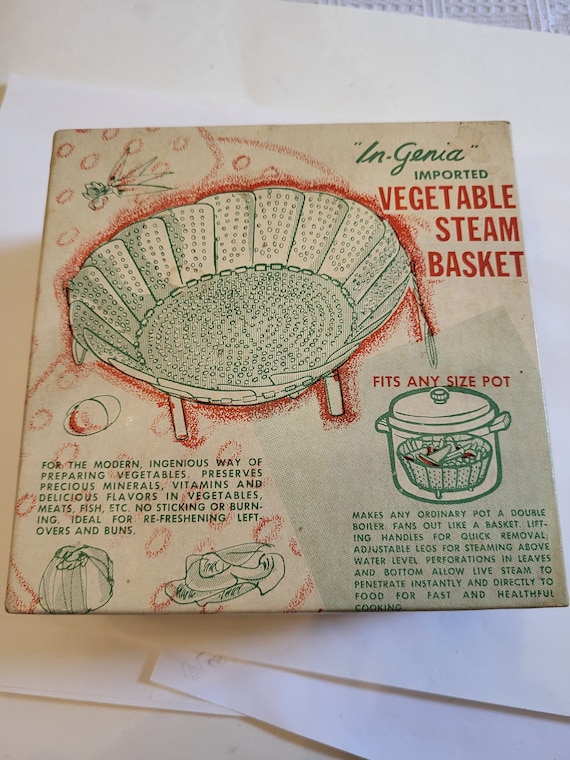The image showcases an old, weathered beige-colored package for a product named the "Ingenia Imported Vegetable Steam Basket." The package features a predominantly green and red color scheme, with "Ingenia" and "Imported" in green text at the top, and "Vegetable Steam Basket" in large red letters beneath. The background appears to be several pieces of paper stacked atop a textured tablecloth.

Illustrated on the package is a colander-like steam basket with flat, perforated surfaces. To the left of this basket is a picture of crudely drawn carrots at the top and an onion at the bottom. Beside the basket illustration, there is a transparent pot outlined in gray, demonstrating how the basket sits inside.

The package includes detailed explanatory text, highlighting the product's features and benefits:

- **Features:**
  - Fits any size pot.
  - Converts an ordinary pot into a double boiler.
  - Fans out like a basket with lifting handles for quick removal.
  - Adjustable legs for steaming above water level.
  - Perforations in the leaves and bottom allow steam to penetrate directly for fast, healthful cooking.

- **Benefits:**
  - Preserves minerals, vitamins, and flavors in vegetables, meats, and fish.
  - Prevents sticking or burning.
  - Ideal for refreshing leftovers in buns.

The overall vintage design, while in good physical condition, emphasizes a modern, ingenious approach to preparing vegetables, marking it as a potentially classic yet functional kitchen tool.